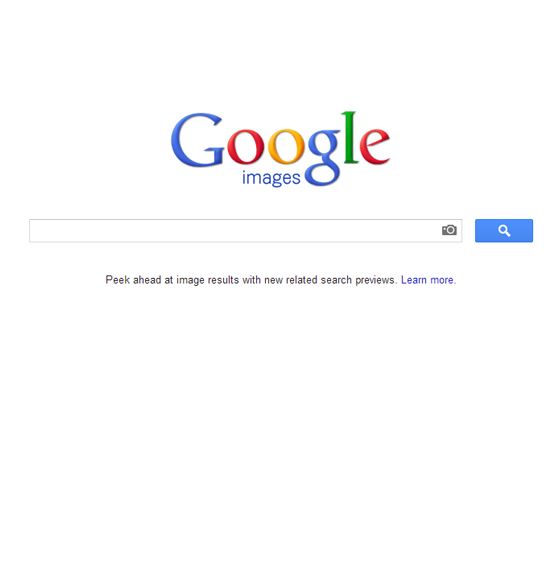The image features a clean, white background with the Google logo prominently displayed at the top. The logo is composed of the letters G-O-O-G-L-E, colored in blue, red, yellow, blue, green, and red respectively. Below the logo lies a rectangular search box, which is flanked on the right by a gray camera icon, indicative of image search functionality. To the immediate right of the camera icon sits a blue search button featuring a white magnifying glass symbol.

Underneath this search section, there's a line of black text that reads, "Peek ahead at image results with new related search previews." To the lower right of this text, "Learn more" is highlighted in blue, signaling it as a clickable hyperlink.

The overall design is minimalistic and intuitive, characteristic of Google's user-friendly interface.